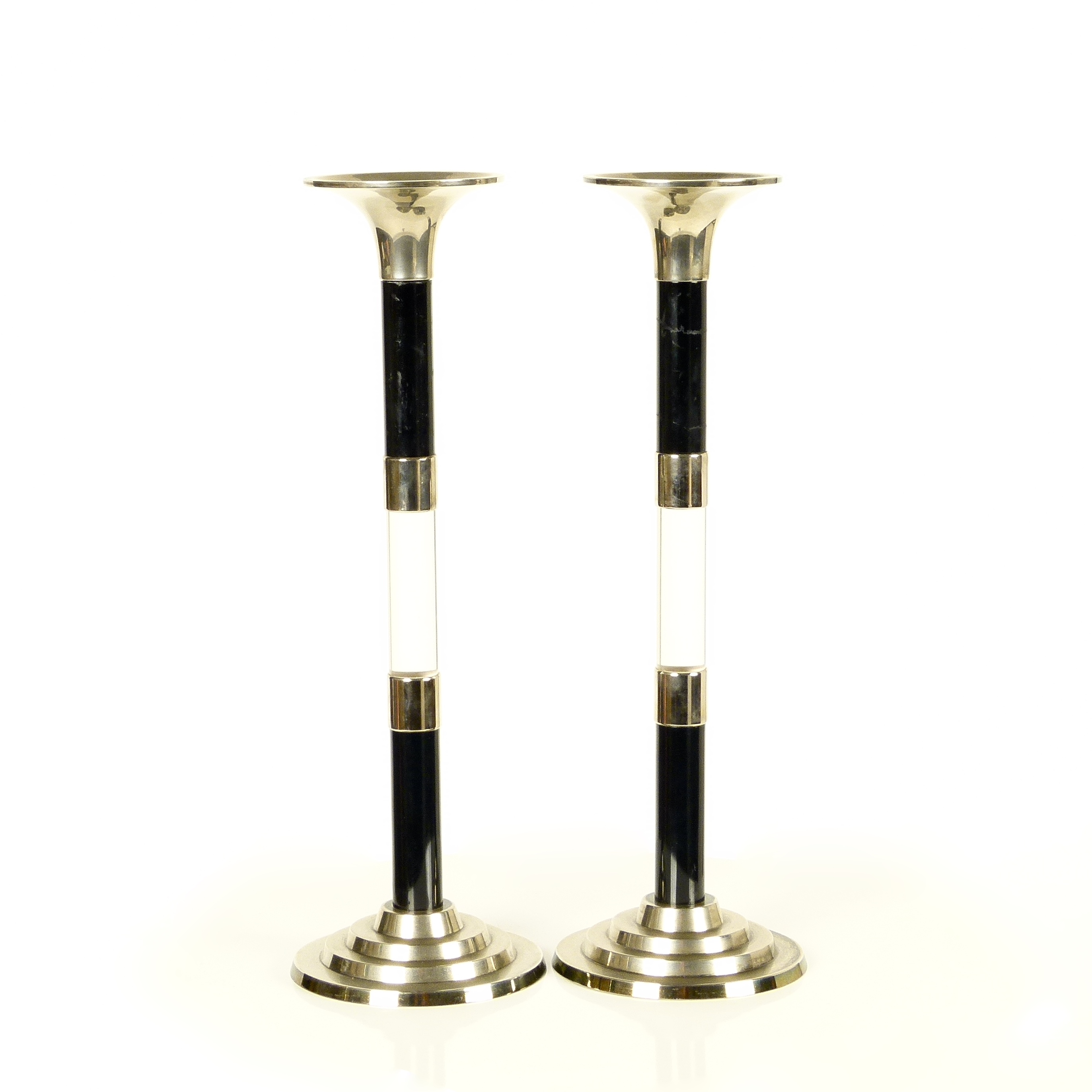The image features two elegant candlesticks, positioned on the left and right sides against a plain white background with a subtle peach tone towards the bottom. Each candlestick stands at approximately four inches tall, with the bases measuring about an inch wide. The bases are crafted from a shiny gold-toned metal, designed in a tiered, circular fashion resembling a set of steps, with four progressively smaller circles ascending towards the central cylinder.

The central cylinder of each candlestick exhibits a sequential pattern of colors and finishes: starting with an inch of glossy black, followed by a small quarter- to half-inch band of the shiny gold metal, then an inch of white, another band of gold, another inch of black, and finally, the tops flare outwards into a flat surface where a candle would sit, capped off in the same lustrous gold metal. The reflective surfaces of both the gold and black sections add a touch of sophistication, while the white band appears potentially luminescent. The minimalist background offers no additional context, drawing full attention to the intricate details and craftsmanship of the candlesticks.